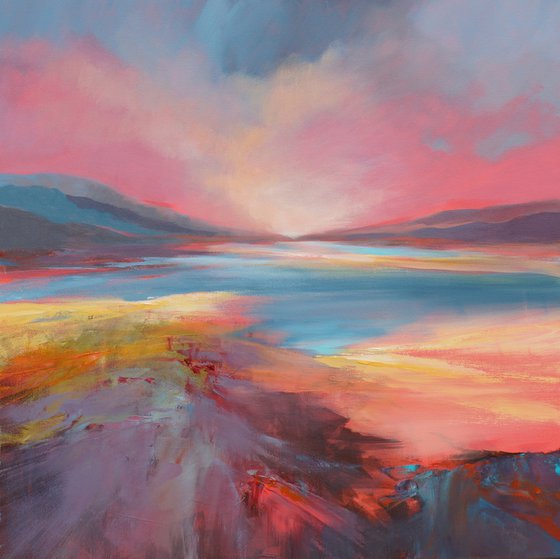This captivating watercolor painting showcases a vivid, colorful landscape depicting a serene and elegant outdoor scene. Dominated by an array of colors, the painting features a contrasting blend of pink, blue, yellow, orange, red, and green. The central part of the image predominantly displays a calming blue, resembling a lake or body of water. Above this, the sky is beautifully marbled with pink hues, suggesting a picturesque sunset. Flanking the water on both the left and right sides are sloping mountain ranges rendered in dark gray and blue tones, giving the scene a sophisticated, almost feminine elegance. Near the bottom left, the colors transition into purple and red, while the bottom right is imbued with blue. The mid-left region also introduces a touch of green, adding to the overall vibrant diversity. Together, these seamlessly blended colors create a harmonious and breathtaking depiction of a tranquil valley framed by majestic mountains, reflecting the awe-inspiring beauty of nature.